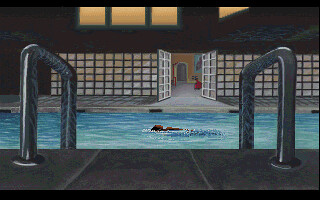In the image, there is an indoor pool setting characterized by a tiled pool deck. The viewpoint of the photograph is through the metal handrails of a ladder, which are installed on both the left and right sides, leading into the pool. The ladder appears firmly affixed to the cement tiles at the pool’s edge. Beyond the focal point of the ladder handles, the pool extends into the background. The water's surface is partially visible and is cut off at both the left and right edges of the image, suggesting a mid-action capture. Additionally, there is an individual swimming towards the left side of the pool, adding a dynamic element to the scene.